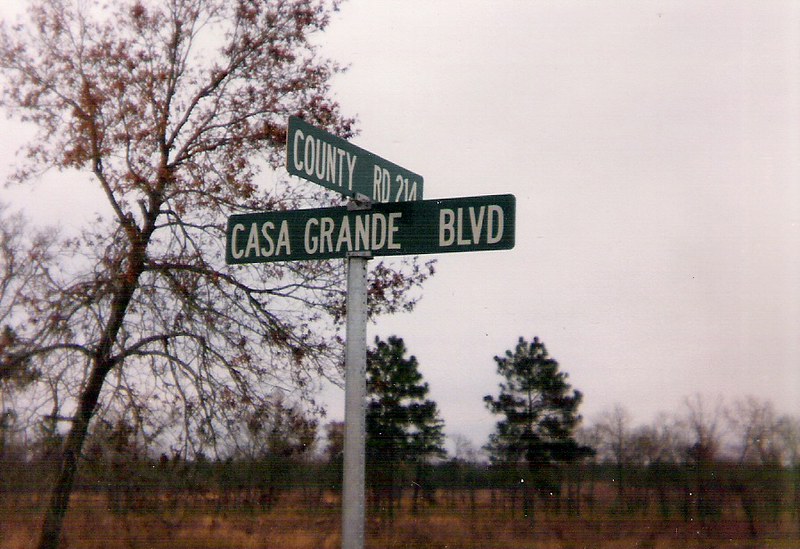This photograph captures a street intersection marked by two road signs, "Casa Grande Boulevard" and "County Road 214." The scene is cloaked under a thick layer of dark clouds, typifying a dreary winter day. In the backdrop, a mix of evergreen trees stands, providing a stark contrast with their rich green and some with brown needles due to the season's harshness. Deciduous trees, stripped of their leaves, add to the wintry ambiance. The grass covering the ground appears yellow and brown, lifeless in the cold weather. Despite being taken in the middle of the day, the overcast sky casts a somber, muted light over the landscape.